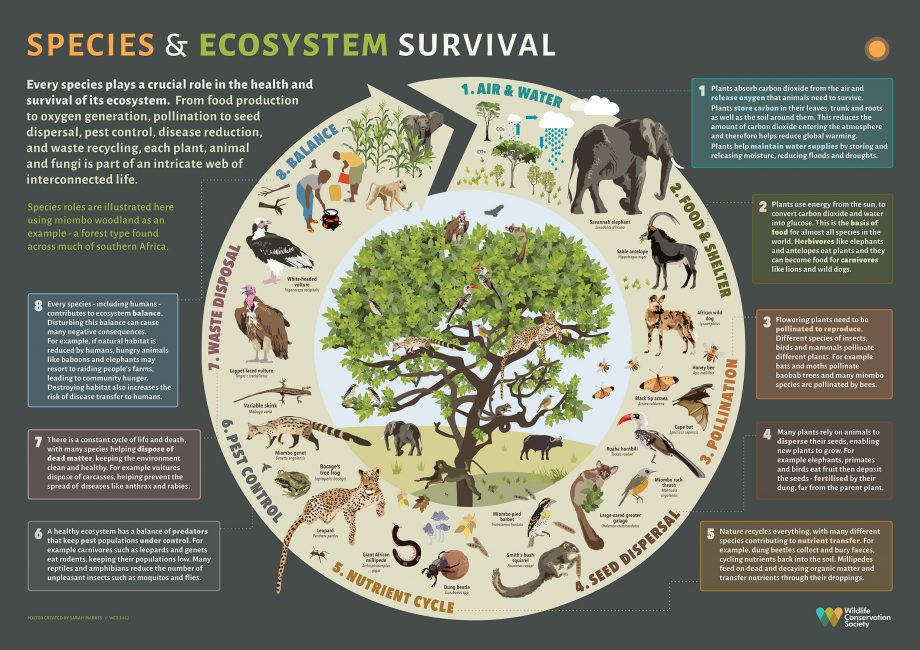The image is a detailed, colorful landscape illustration titled "Species and Ecosystem Survival," presented in a circular diagram format. The central focus is a green tree surrounded by various animals, symbolizing different ecological functions. The circle is divided into eight distinct sections: Air and Water, Food and Shelter, Pollination, Seed Dispersal, Nutrient Cycle, Pest Control, Waste Disposal, and Balance. Each section is populated with specific species associated with these functions, such as elephants for Air and Water, gazelles for Food and Shelter, bats, butterflies, and bees for Pollination, squirrels and birds for Seed Dispersal, millipedes and insects for the Nutrient Cycle, and leopards and lizards for Pest Control. The backdrop is a dark gray or black poster with small explanatory text on either side of the diagram, providing further details on each ecological category. Throughout the circular motion, the diagram illustrates the interconnectedness of various species—ranging from elephants, goats, rats, birds, leopards, and cheetahs to vultures, eagles, and monkeys—in maintaining ecosystem balance and survival.